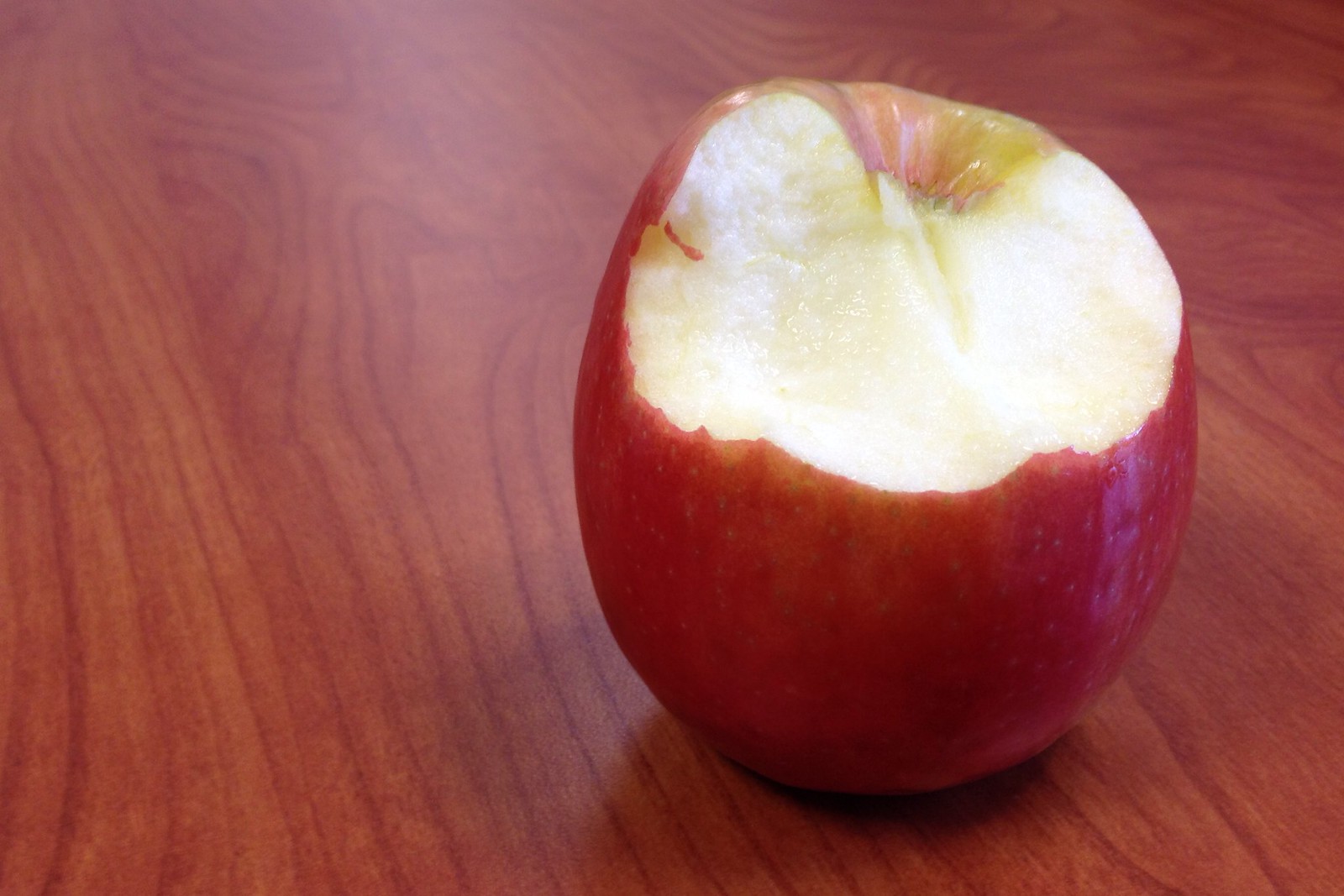A red apple, reminiscent of the one from Snow White, sits slightly off-center towards the bottom right of a wooden table, which serves as the entire background. The apple has been partially eaten, specifically around the top where the stalk once was, suggesting someone who possibly even consumes the core. Significant bruising is visible on the left side of the apple, along with some minor dings. Though the exposed interior of the apple has started to brown, it is still relatively fresh, indicating it was bitten into not long ago.